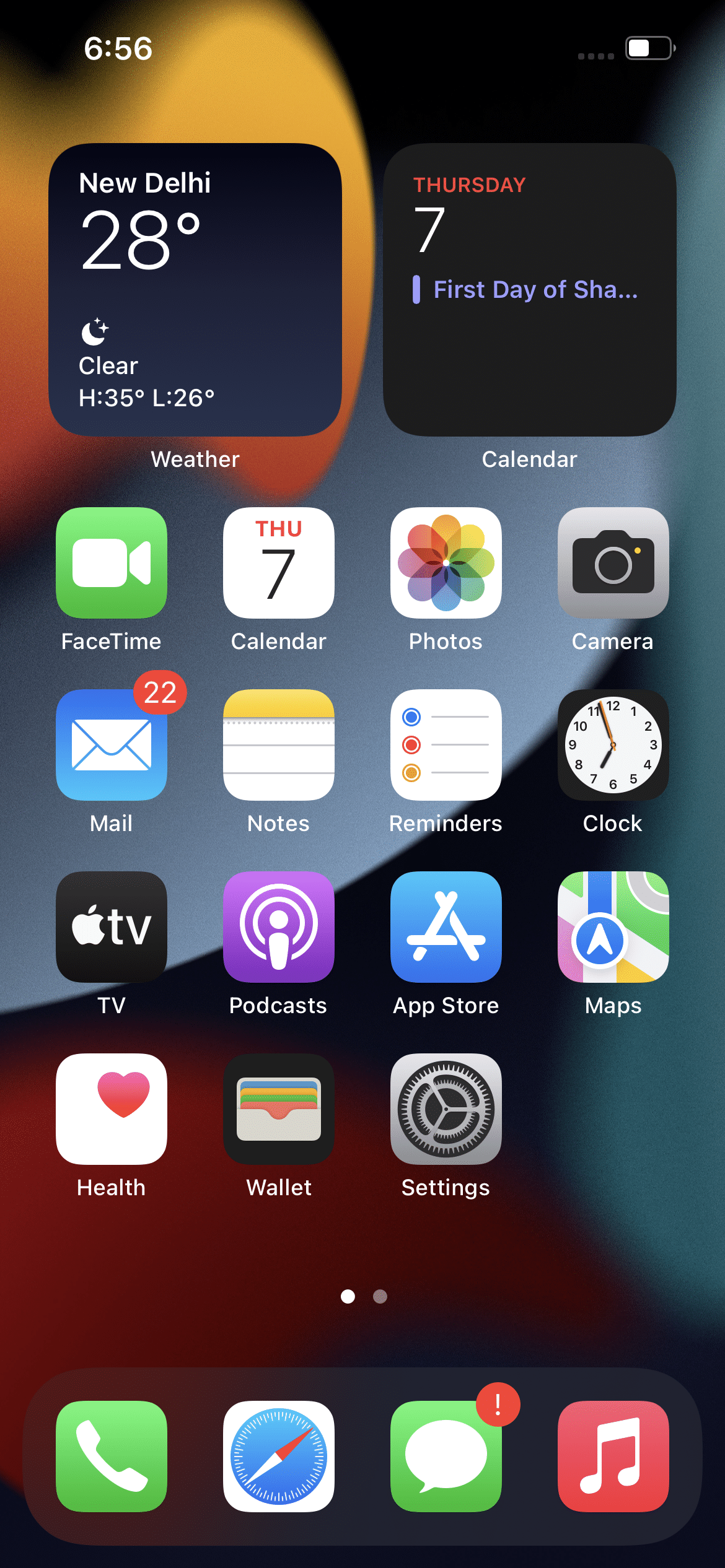A vertical image captures the home screen of a smartphone, displaying a variety of app icons against a blurred background. The background features a gradient of warm and cool tones, with an orange blurry spot in the upper left corner, grayish, faintly glowing lights scattered across, and a reddish circular blur towards the bottom.

On the top left, the time is displayed as 6:56, while the top right shows the battery icon. Below the status bar, two widgets are visible. The first widget on the left provides weather information for New Delhi, showing a current temperature of 28°C, clear conditions, and a forecasted high of 35°C and low of 26°C for Thursday. The second widget on the right reads "Thursday the 7th, first day of Shah…” with the end cut off, alongside a calendar icon.

Beneath the widgets, an array of app icons includes:
- Top row: FaceTime, Calendar, Photos, Camera
- Second row: Mail, Notes, Reminders, Clock
- Third row: Apple TV, Podcasts, App Store, Maps
- Bottom row: Health, Wallet, Settings 

At the very bottom of the screen are the dock icons for Phone, Safari, Messages (indicating a pending message), and Music. There's an indication to scroll to additional pages of apps, but these are not visible in this image. The setup reflects an organized, yet personalized digital space, with essential applications at the user's fingertips.